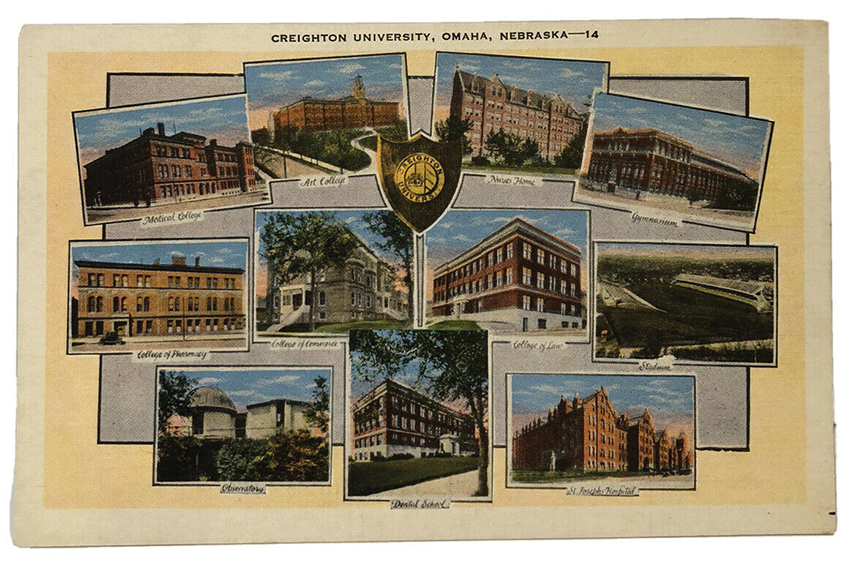This is a color postcard featuring Creighton University, Omaha, Nebraska, -14. The postcard is framed with a white border, inside which is a series of smaller rectangular images of various university buildings. There are 11 such pictures, arranged in rows, all set against a layered background of gray, black, and yellow-tan. At the top of the postcard, in black ink, it reads "Creighton University, Omaha, Nebraska-14."

In the center of the postcard is a shield-shaped icon with a brown exterior and a yellow circle inside that also reads "Creighton University." Underneath each building image is a small black script caption, although they are quite difficult to read due to their size. Legible captions include names like "Art College," "Medical College," and "College of Pharmacy." The intricate layering of borders and the multiple images provide a detailed and informative visual representation of the university's campus architecture.